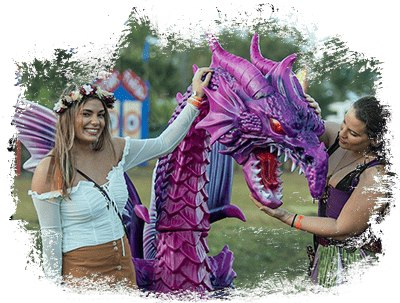In the photograph, two young women are posing playfully with a fierce-looking purple dragon sculpture at what appears to be an outdoor fair or carnival. Both the women are dressed in festive, summery attire: the woman on the left sports off-the-shoulder white top, a khaki skirt, and a garland of flowers in her blonde hair, while the woman on the right wears a purple corset-like tank top, green skirt, and has dark brunette hair. They stand on green grass, with out-of-focus trees and an indistinct sign in the blurry background.

The dragon sculpture, positioned taller than the women, features intricate details including purple wings, a long neck, red eyes, pointed teeth, a fierce tongue, and fin-like purple ears. It stands between them, its long snout and menacing expression adding an element of fantasy to the scene.

The photograph has been edited in post-processing, giving the edges an irregular, smeared appearance, possibly through an eraser effect in Photoshop. Despite the background blur, the vivid details of the women and the dragon are sharp, capturing their enjoyment and the whimsical atmosphere of the event.